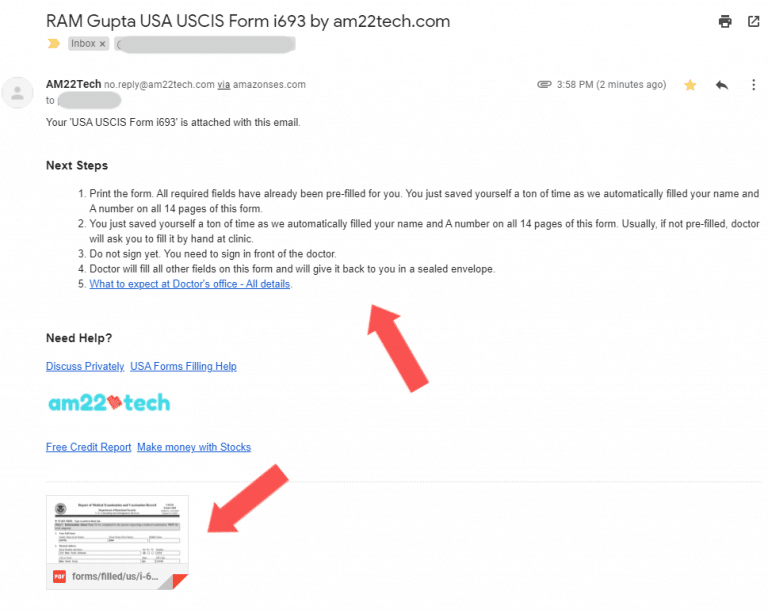Screenshot of an email from Ram Gupta (USCIS Form I-693) sent by am22tech.com. The "To" section of this email is grayed out. The main body of the email is titled "Next Steps" and contains a list of five steps. The fifth step, "What to Expect at the Doctor's Office," is highlighted in blue, indicating it is a clickable link. A red arrow points to the "Next Steps" section in the email. Another red arrow indicates an attachment listed at the bottom of the email. At the bottom, there's a business logo that reads "am22tech" in teal color.